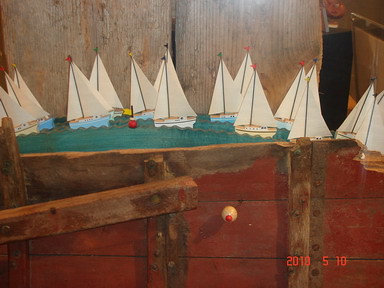This 2010 dated color photograph captures a detailed diorama set inside what appears to be the side of an antique wooden wagon, identifiable by its red-painted slats and upright stays. The centerpiece is a vibrant depiction of a river, its greenish-blue waves carved and painted from wood, hosting a flotilla of intricately crafted miniature sailboats. There are approximately 18-20 sailboats, each adorned with white sails and small, differently colored pennants—red, green, and dark blue—at their tops. The boats themselves vary in color, including shades of blue, white, and ivory. Among the sailboats is a small red buoy, adding to the realism of the scene. This elaborate display captures the essence of vintage craftsmanship and maritime charm.